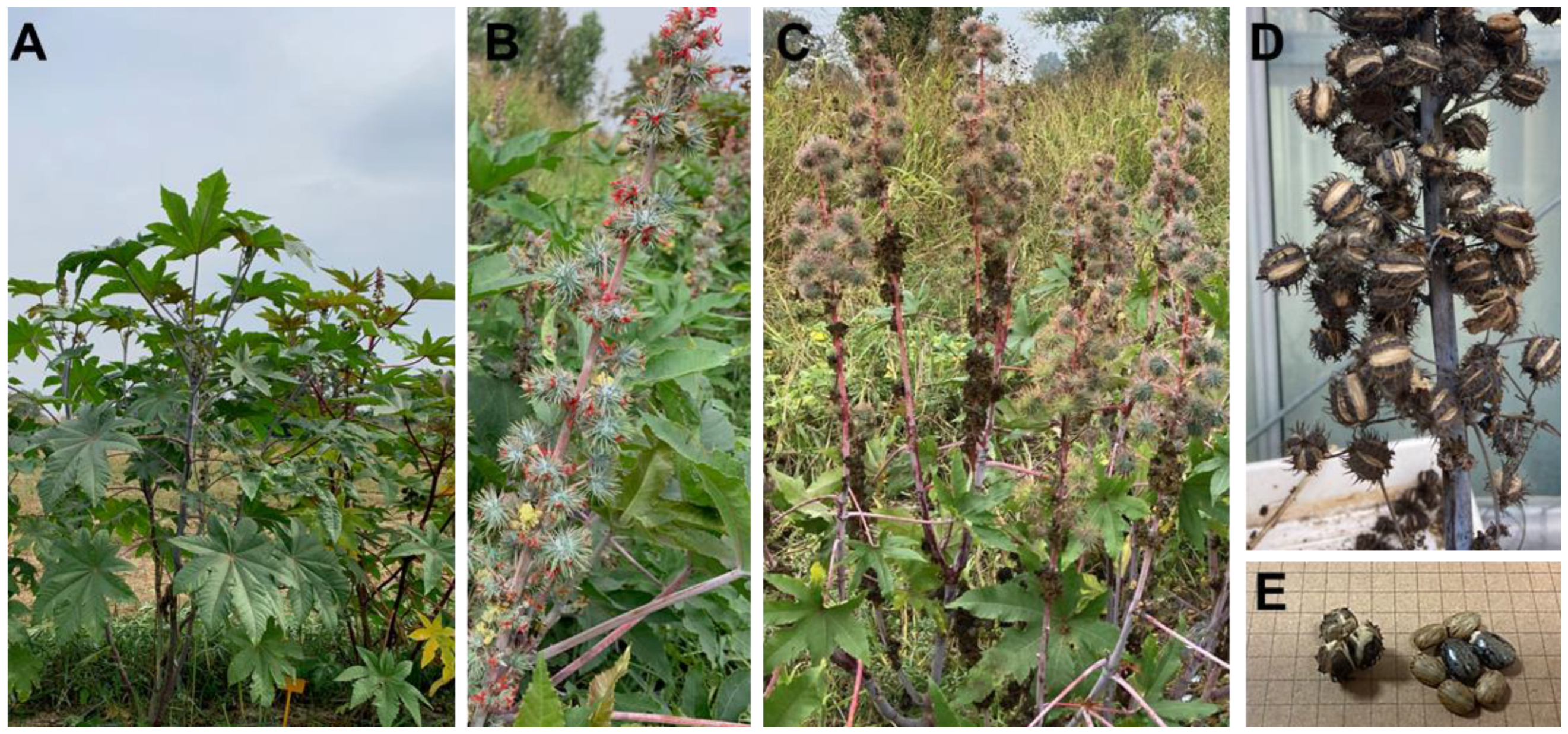The image presents a detailed collage of five plant-related pictures, labeled A, B, C, D, and E. 

- **Image A**: This section features a foreground of green weeds with leaves, set against a backdrop of grass and a field possibly covered with hay. The sky above is partly cloudy, adding a natural ambiance to the scene.
- **Image B**: Centered around a flowering weed, this plant showcases a colorful array with pink, yellow, light green, and possibly red hues on its buds.
- **Image C**: Depicts round, light green structures that resemble cotton weed, growing from branched stems, surrounded by green leaves.
- **Image D**: This might be an indoor shot, highlighting a grayish stem or trunk with round, striped-off green and light yellow formations, resembling seeds or unique growths.
- **Image E**: Contains oval-shaped objects on a light tan tiled surface, which could be seeds or stones, exhibiting colors like light tan, gray, pink or red, yellow, and very light blue.

Overall, the collage captures different plants and their elements in various stages and settings, from lush weeds to detailed seeds and flowering buds, with a spectrum of colors including green, yellow, pink, red, and many others against natural and indoor backgrounds.